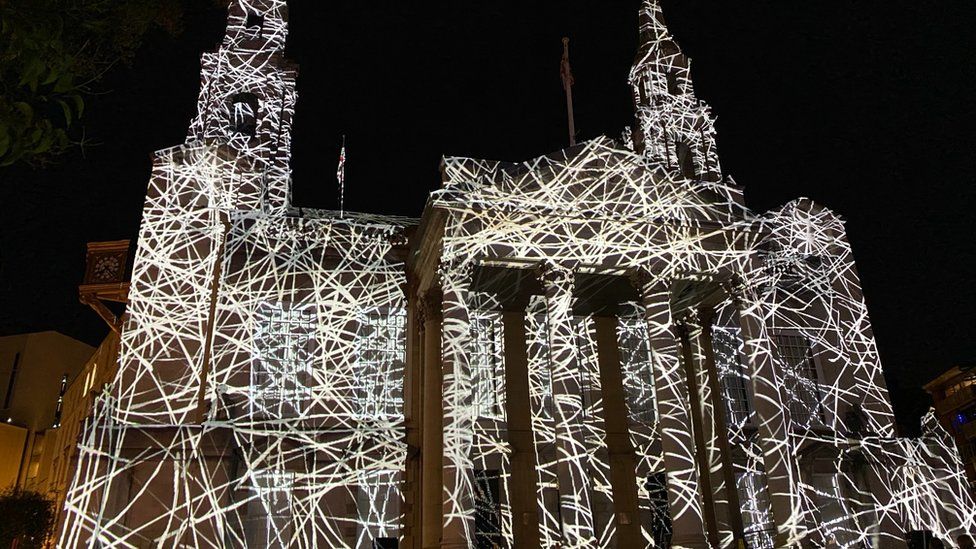This is a nighttime photograph taken outdoors, depicting a striking structure completely enveloped in white lines that resemble strings, tape, or possibly even paper. The building, which appears to be a church, is outlined by these luminous white strings that cascade down from its two side towers, creating a striking visual effect akin to being wrapped in light. The structure's front towers or pillars, four in total, stand prominently illuminated against the pitch-black sky, adding to the surreal appearance. To the left of the building, a lit window can be seen in the background, suggesting that part of the building might be under construction. The entire scene is bathed in an eerie glow from these thin, continuous lights, creating a mysterious and captivating image.